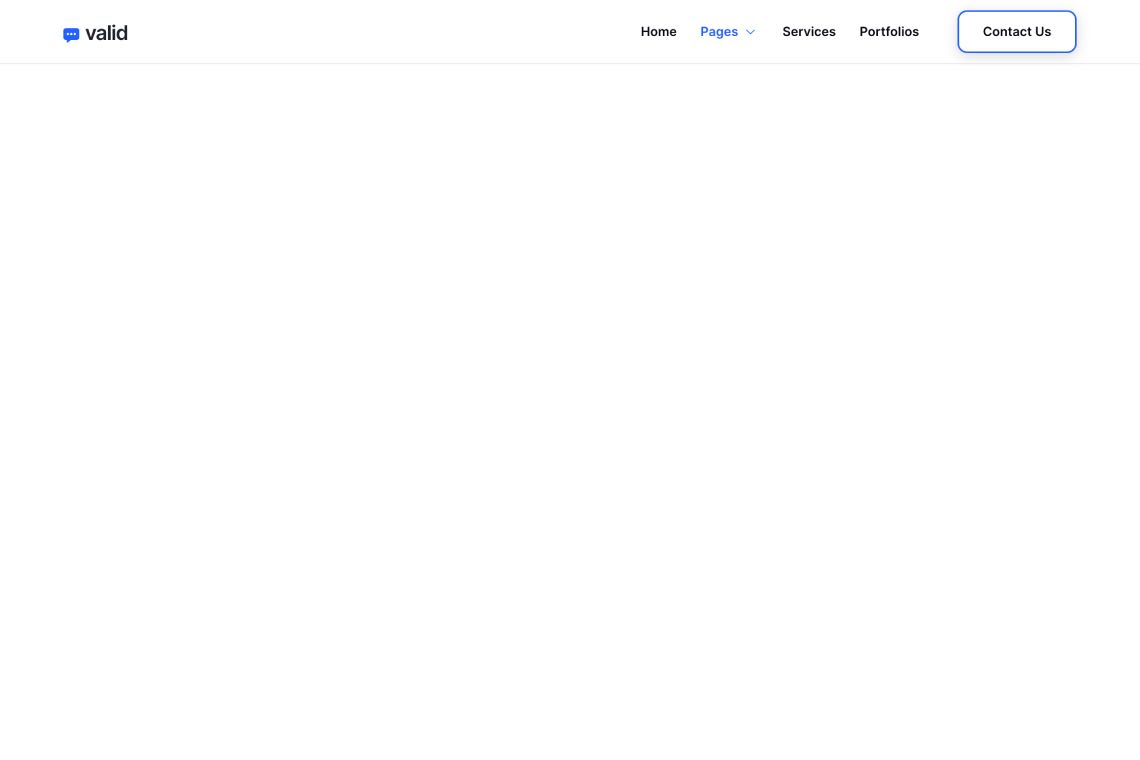The screenshot depicts a minimalist section of a website interface, primarily showcasing the elements of its top navigation bar. Against a plain white background, a light gray line delicately outlines the upper edge, demarcating the start of the webpage. 

In the top left corner, a blue chat logo featuring three white dots is visible, adjacent to the lowercase word "valid" written in black. This visual suggests the website's branding. Proceeding rightward along the navigation bar, the menu items are laid out in the following order: "home," "pages" (highlighted in blue to denote the active page), "services," and "portfolio." The series concludes with a prominent "contact us" button, outlined in navy blue. The sparse design of the capture leaves the web page's content and purpose to the imagination.